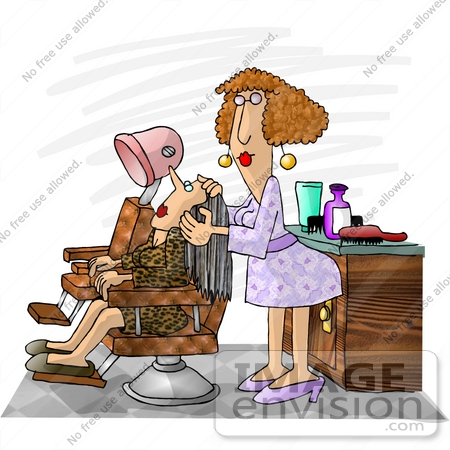In this vibrant, cartoon-style illustration, a woman with graying hair adorned with white streaks is seen reclining in a salon chair, wearing a cheetah-print dress and brown shoes. She has red lipstick on, adding a pop of color to her look. Standing behind her is the hairstylist, a woman with short, curly light brown hair, dressed in a light purple dress adorned with white and purple flowers, and cinched at the waist with a purple belt. She too has red lipstick and is accessorized with dangling gold ball earrings.

The salon setting is detailed with a second, unoccupied chair that features an overhead hairdryer, and a brown cabinet positioned behind the stylist. This cabinet, which has a gray top and gold handles, is topped with various hairdressing tools including a red-handled brush, a black comb, a green squeeze tube, and a couple of bottles in blue and purple hues. The room is primarily decorated in brown tones, adding warmth to the scene. There's faint watermark text throughout the image that reads "no free use allowed," and at the bottom right corner, the website "imageinvision.com" is subtly inscribed.